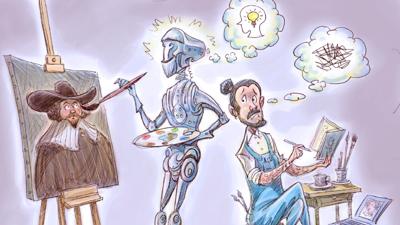In this horizontally rectangular cartoon image with a light purple background, a vivid scene unfolds on the left side with a robot diligently painting at an easel. The robot, equipped with a brush and palette, is creating a detailed portrait of a man dressed in colonial attire—a big brown hat, a brown coat, and a large white collar. Above the robot, a thought bubble featuring a head with a light bulb signifies a eureka moment or an inspired idea. To the right, a human artist, wearing overalls and a white t-shirt, sits on a low stool. This artist looks perplexed or irritated, gazing at the robot as he sketches in a book placed on a small table that holds paintbrushes and a cup. The adjacent thought bubble above the human displays jagged lines, indicating frustration and lack of inspiration. This scene juxtaposes the creative, efficient robot against the struggling human artist, potentially commenting on the evolving dynamic between artificial intelligence and human creativity.